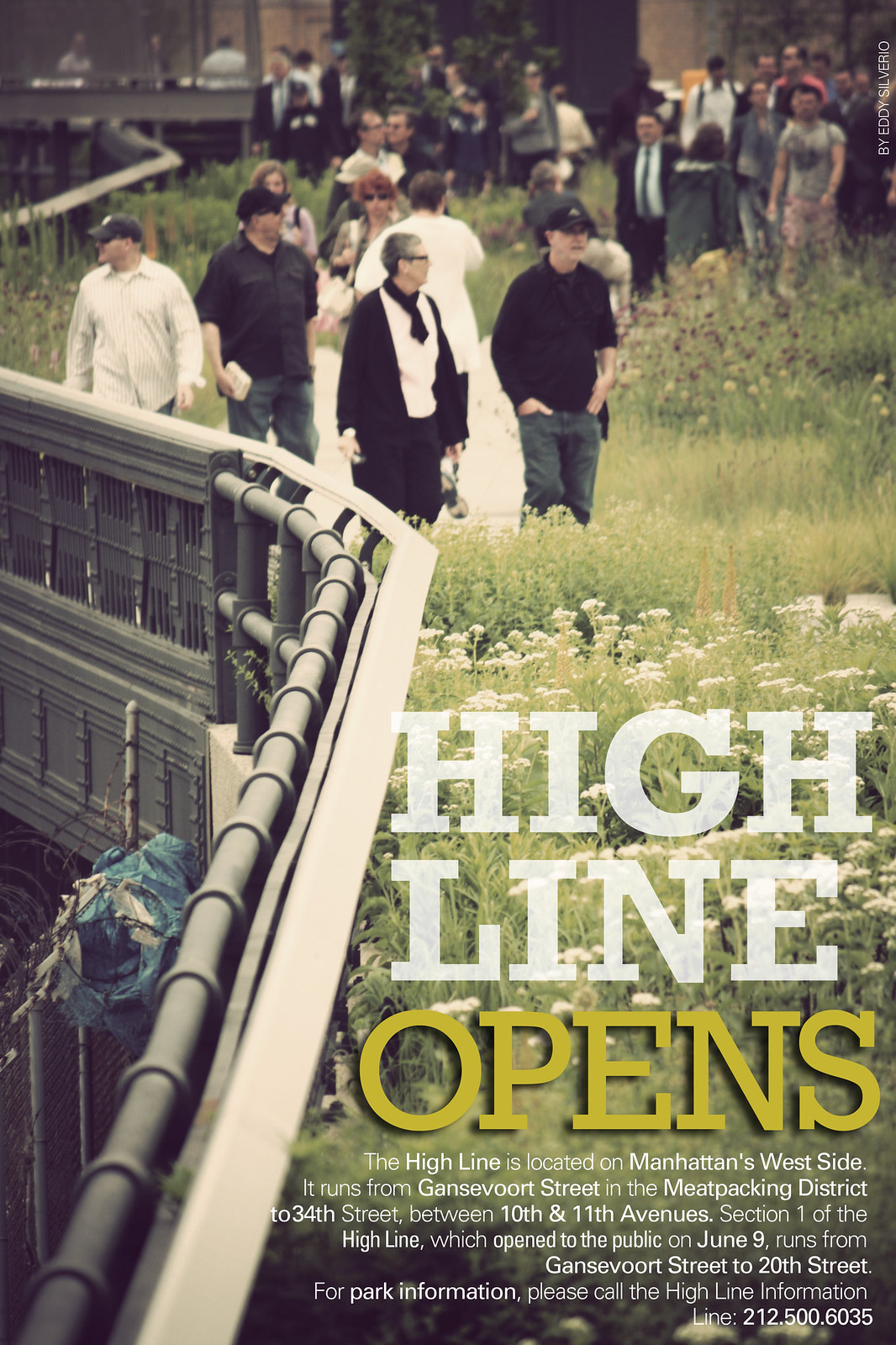The flyer features a vibrant image of a group of people standing in a field on a bridge, surrounded by blooming white, deep red, and yellow flowers. These individuals, some dressed in black and white, highlight the community's engagement with this urban park. Dominating the lower third of the flyer on the right side, bold white capital letters announce "HIGH LINE," followed by "OPENS" in striking puce green. The detailed text provides essential information, stating that the High Line is situated on Manhattan's west side, stretching from Gansevoort Street in the Meatpacking District to 34th Street, between 10th and 11th Avenues. It specifies that Section 1 of the High Line, which became accessible to the public on June 9th, extends from Gansevoort Street to 20th Street. For more details, visitors are encouraged to contact the High Line information line at 212-500-6035. The imagery and text collectively serve to invite the public to explore and enjoy this elevated park.